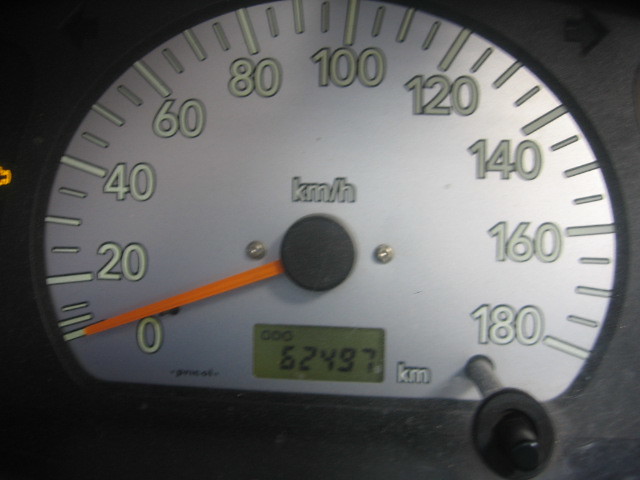A detailed description of the image:

A speedometer with a range from 0 to 180 km/h is prominently displayed. The outer ring of the speedometer features tick marks at intervals of 20 (0, 20, 40, 60, 80, 100, 120, 140, 160, 180). Below the tick marks, the units "KM-H" are clearly labeled. The speedometer's face is mainly silver with a surrounding black rim. At the center is a large black circle, from which an orange needle extends, currently pointing towards 0. The background of the speedometer is predominantly silver, contrasting with the black elements, making the details stand out vividly.